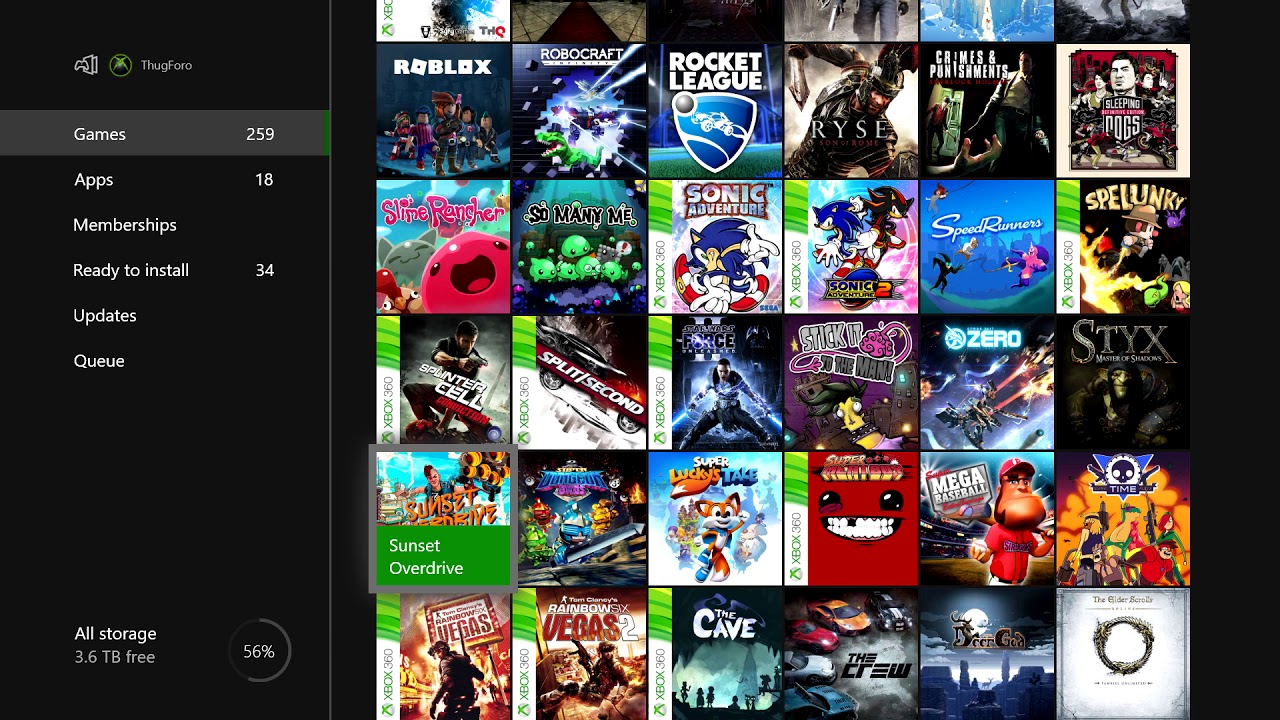In this image, we observe a vibrant collection of video game icons displayed in a grid format, specifically a 5x6 block array, making up a total of 30 game icons. Each icon is colorful and easily recognizable, representing a variety of popular video games. On the left side of the screen, there is a sidebar featuring detailed categorization and storage information. It indicates the following:

- Games: 259
- Apps: 18
- Memberships: Ready to Install 34
- Updates Queue

Furthermore, at the bottom of the sidebar, storage information is provided, indicating all storage at 3.6 TB with 56% of it either free or used.

Notable game icons visible in the image include:
- Roblox
- Rocket League
- Sleeping Dogs
- Sonic Adventure
- Zero Sticks
- Spelunky
- Super Lucky's Tale
- Rainbow Six Vegas 2
- The Cave
- The Crew
- The Elder Scrolls Online
- Sunset Overdrive

The background is predominantly black, which contrasts well with the white text and the colorful game icons, making them stand out clearly. The detailed text and array of game icons give a comprehensive view of the user's gaming library.